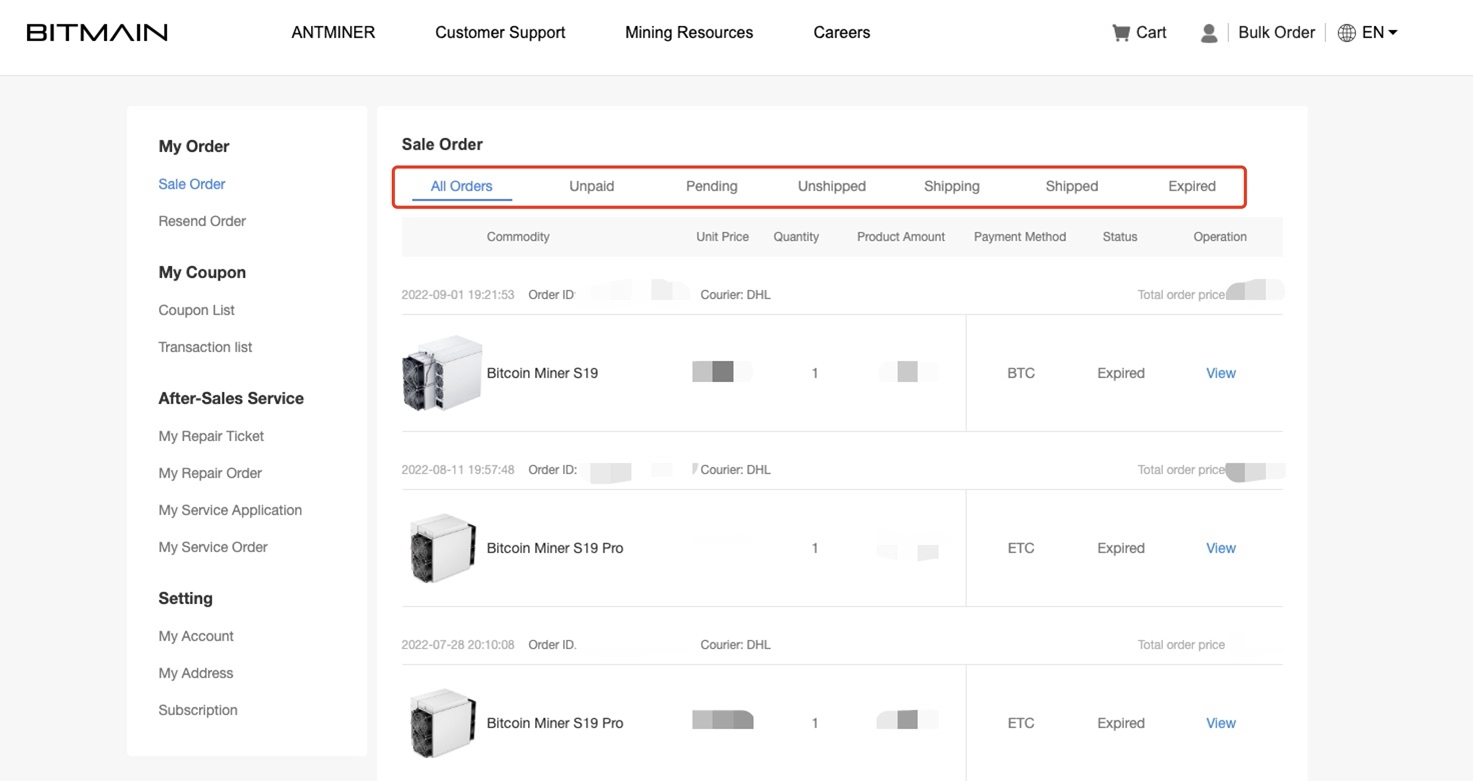Screenshot of the Bitmain website interface. 

The website header prominently displays the Bitmain logo on the left, followed by navigation options: Antminer, Customer Support, Mining Resources, Careers, Cart, Profile Icon, Bulk Order, and a globe icon labeled "EN" indicating language options.

On the left sidebar, a vertical menu includes options such as:
- My Order
- Sale Order (highlighted in blue)
- Resend Order
- My Coupon
- Coupon List
- Transaction List
- After Sales Services
- My Repair Ticket
- My Repair Order
- My Service Application
- My Service Order
- Setting
- My Account
- My Address
- Subscription

In the main content area, the heading "Sale Order" is prominently displayed. A red box highlights a horizontal tab menu featuring categories:
- All Orders
- Unpaid
- Pending
- Unshipped
- Shipping
- Shipped
- Expired

Beneath this menu, column headers indicate details for each order:
- Commodity
- Unit Price
- Quantity
- Product Amount
- Payment Method
- Status
- Operation

Below these headings, a list of Bitcoin miners is displayed, giving users the option to view different products.